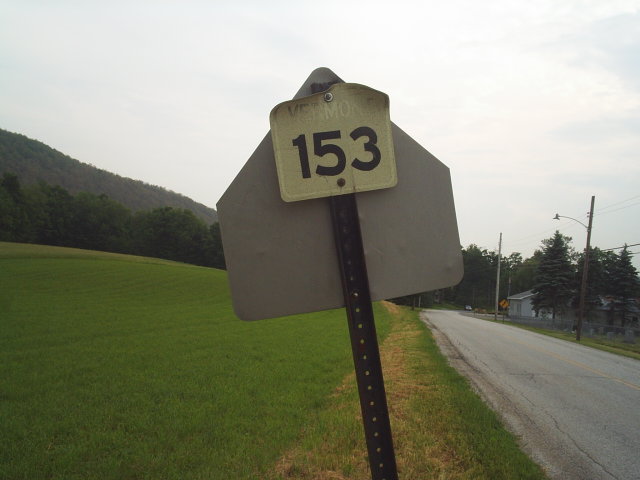The image features the backside of a large, gray street sign prominently in the foreground. Attached to this larger sign is a smaller, old, and bent white square sign that appears to be aged and worn. The smaller sign has the word "Vermont" faded with time and the number "153" clearly visible in black. The backdrop includes an expansive meadow of green grass leading to a gravel road. On the right side of the image, a small house is nestled among trees, light poles, and power lines. The left side reveals a dense cluster of trees and a mountainous range in the distance, all under a hazy sky. The overall scene exudes a rustic and serene countryside atmosphere.